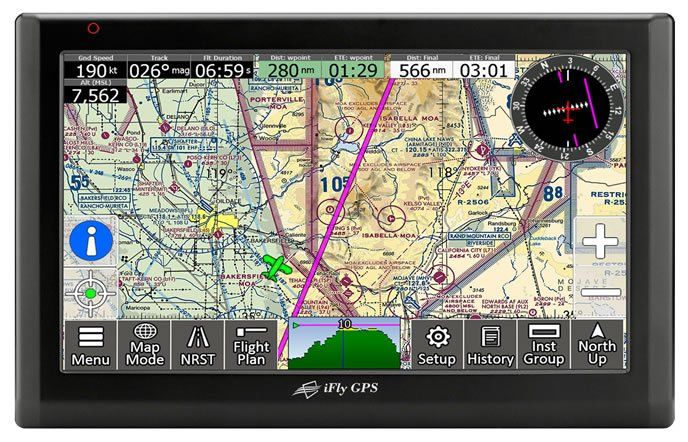This image displays a rectangular-shaped iFly GPS device, framed by a gray border, prominently featuring a screen that covers most of its surface. Central to the screen is a multi-colored map showcasing various routes and highlighted roads, with degrees and coordinates visibly marked. At the top of the display, there are gauges indicating an altitude of 190, a magnetic heading of 026 degrees, and a specific time of 6:59, with the GPS system registering 7,562 feet. In the upper right corner, a black compass set within a gray border is visible, accompanied by plus and minus icons just below it. The lower section of the screen displays clickable tabs or toggle switches for different modes, including options like map mode, NRST, flight plan, setup, history, INST group, and north up with an upward arrow. To the left side, there is a blue information button with a white 'i'. Additionally, numerical data is present, showing 280 NVM and 0129 in green, and 566 NVM and 0301 in white. The bottom center of the device prominently features the "iFly GPS" logo. This detailed depiction underscores that the GPS system is designed for aircraft navigation.